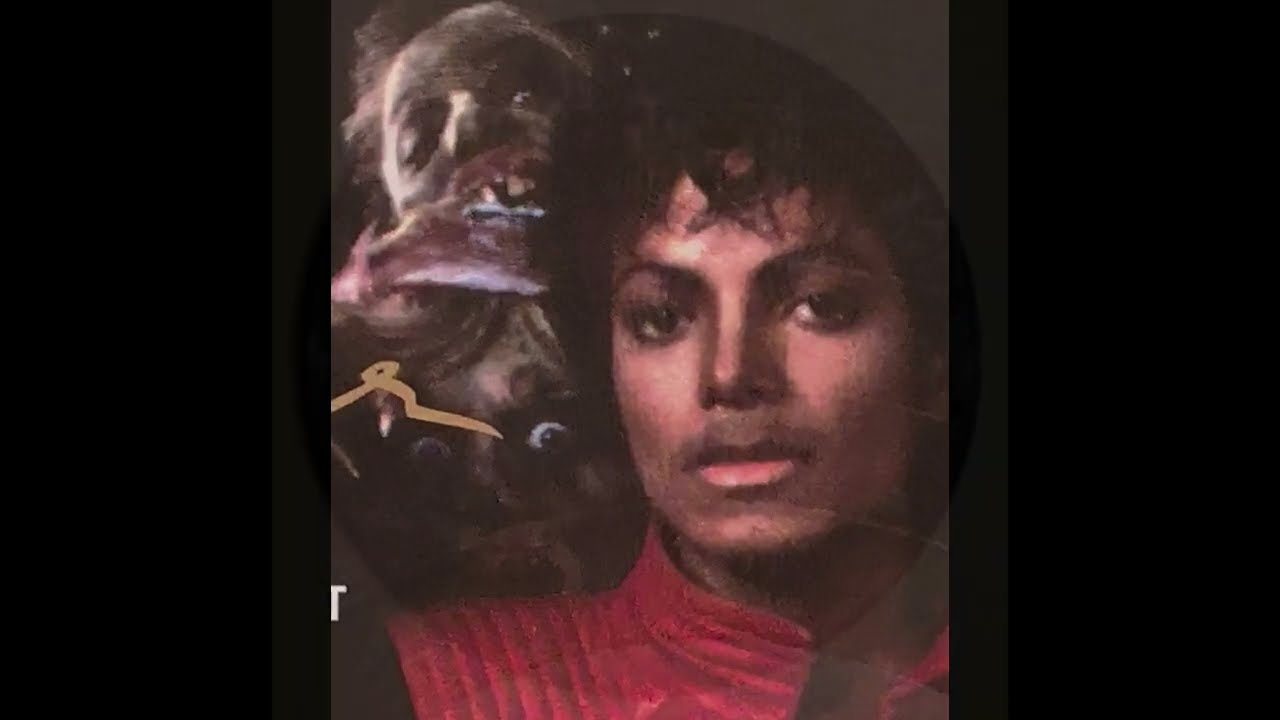This detailed image features Michael Jackson from the iconic "Thriller" music video. He stands confidently at the center, staring directly at the camera. His characteristic dark curls frame his face, and he's dressed in an open, red leather jacket that reaches to his sleeves, giving it a vest-like appearance. Flanking him are two eerie figures: to his left, a zombie-like creature with wide-open blue eyes and disheveled, dark hair appears frightened, casting a spooky gaze at the viewer. Higher above, another monstrous face leans back with an open mouth, displaying jagged, broken teeth and a partially bald head. This chilling vignette, placed in a circular frame against a black background, perfectly encapsulates the haunting essence of the "Thriller" video.